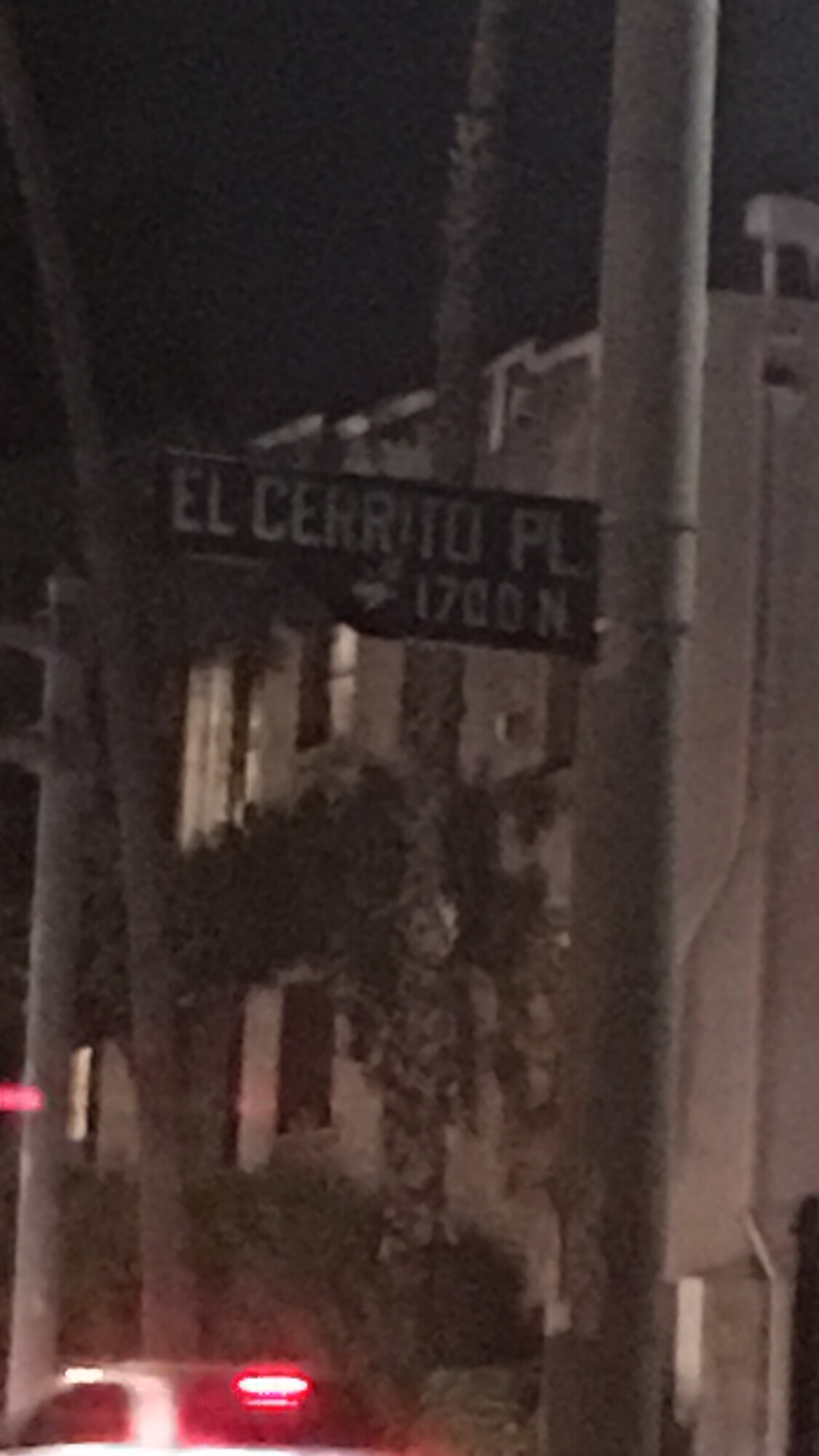The image captures a nighttime street scene focused on a vertical street sign attached to a metal pole, displaying "El Cerrito Place" and "1700 N." The environment is dark, causing some blur, but the sign is distinct and central to the composition. Rising from the ground are the trunks of tall palm trees, and in the backdrop, a sizable building with windows and surrounding bushes are visible. In the bottom left corner, a car with its brake lights on casts a red glow, partially illuminating the scene.